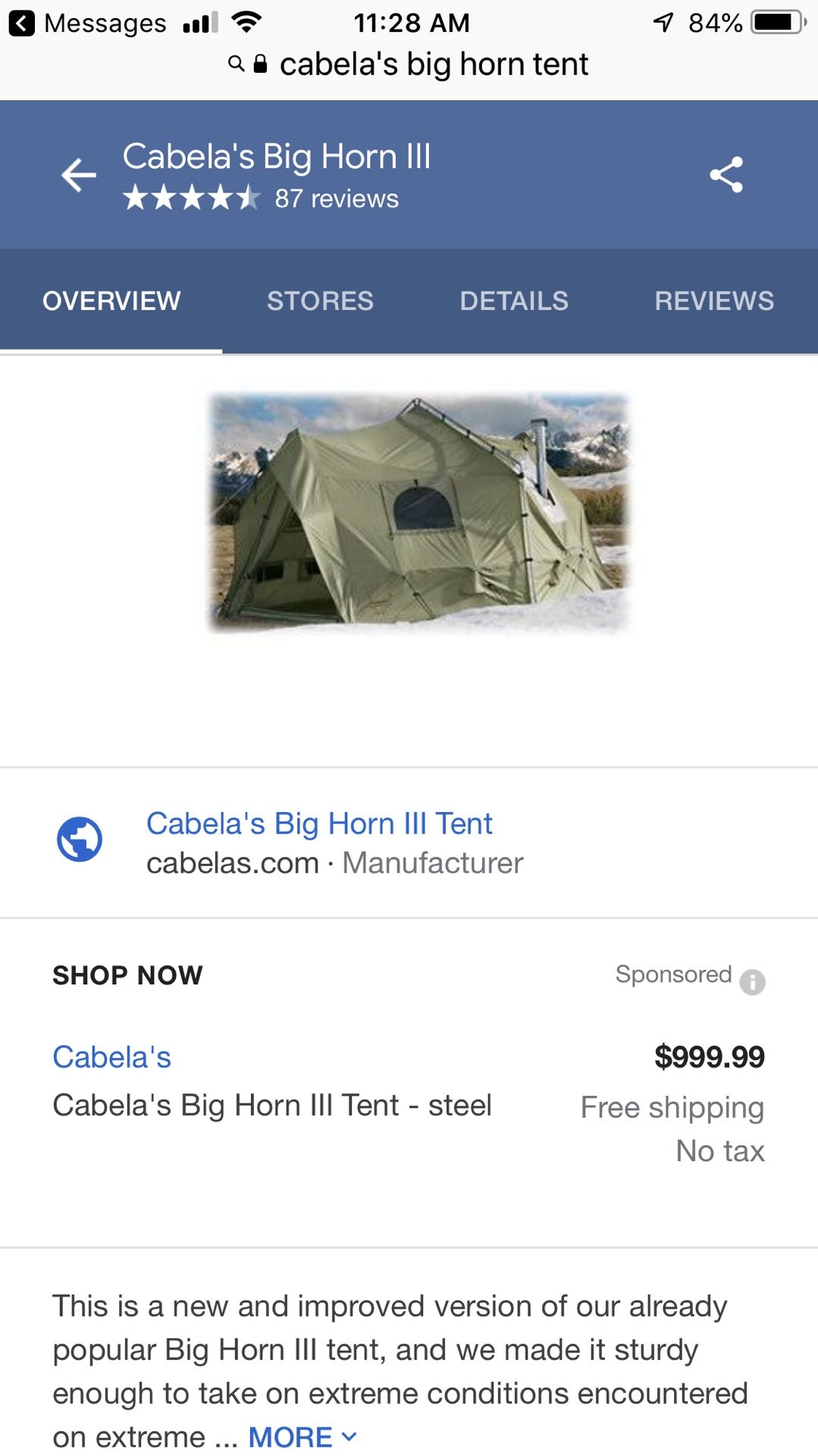Displayed is an app interface showcasing a product listing for the "Cabela's Big Horn III" tent. The tent is large and appears designed to accommodate multiple occupants, featuring a complex and sturdy construction. It’s listed with a price tag of $1,000, boasting free shipping and no tax. Described as a new and improved version of the popular Big Horn III model, this tent is engineered to endure extreme conditions. The tent's color scheme combines a dull green with hints of beige, giving it a rugged look. Above this product listing, the app also features tabs for Stores, Details, and Reviews, although the exact nature of the website remains unspecified.